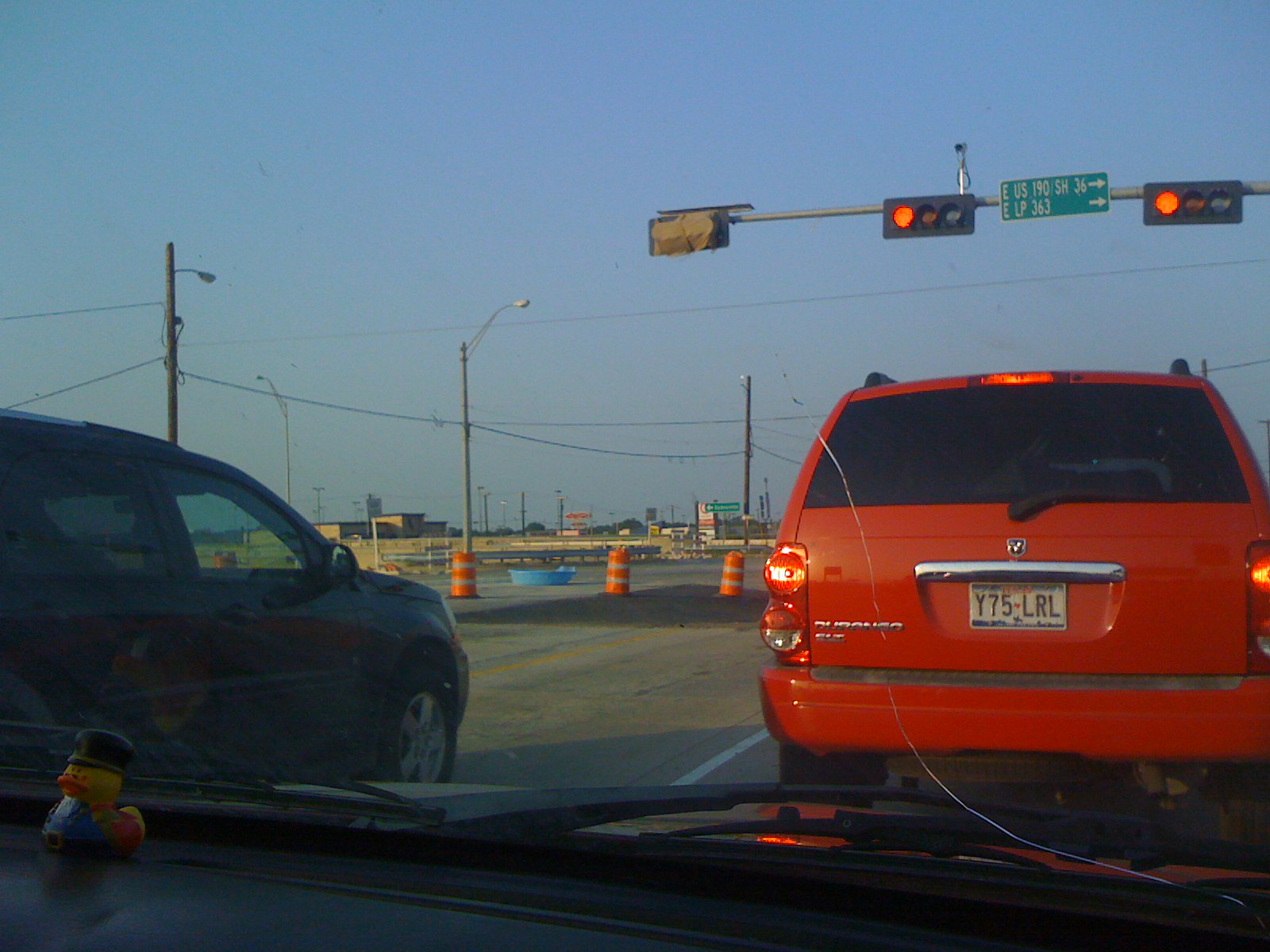The image captures a scene of traffic viewed from inside a car. Through the cracked windshield extending from the bottom right towards the center, a small yellow toy duck wearing a black hat is visible on the dashboard. The vehicle is stopped at a red traffic light, evident by the two red lights at the top right of the image. Ahead is a red Dodge Durango SUV with a Texas license plate reading Y75-LRL, and to the left, there's a black SUV. Overhead, a green road sign reads "East US 190 SH 36" and "East LP 363," indicating directions with right arrows. The sky is clear and blue, and scattered orange traffic cones and some businesses are visible in the distance. The flat landscape is punctuated with light posts and additional cars also waiting at the intersection.